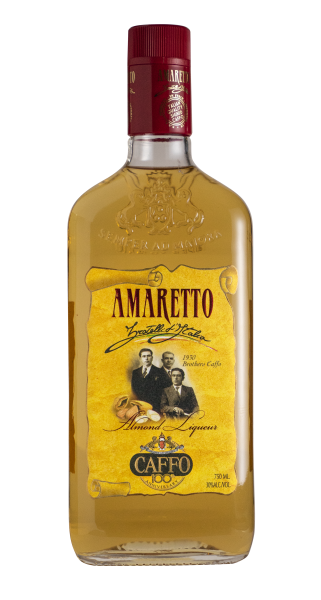This image features a vintage-style bottle of liquor with a golden-hued amaretto inside. The bottle is crowned with a burgundy screw-on cap, inscribed at the top. The bottle is see-through, revealing the liquor within. A distinctive engraving sits at the top of the glass, and below it is a yellowed label designed to resemble aged paper. The label prominently displays the word "Amaretto" in red lettering, with additional descriptive text indicating it is an almond liquor. The label also includes a signature and a black and white photograph of three men, two standing and one seated. Beneath the image of the men, the label reads "CAFFO," and the bottle holds 750 milliliters of the liquor. The background of the image is entirely white, giving the bottle a clean, standout appearance suitable for a website display.